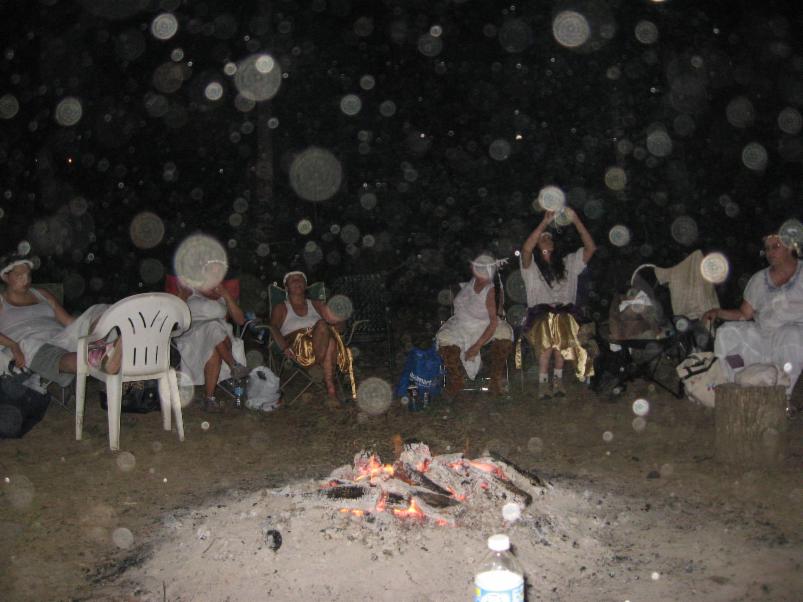The image captures a nighttime beach party centered around a dying campfire, its embers glowing faintly in the sandy soil. The scene is dotted with water droplets on the camera lens, creating scattered white speckles across the photograph, possibly from rain or beach spray. Surrounding the campfire, a group of predominantly women lounge in various chairs. The woman on the far left has her feet propped up and cannot be seen clearly. To her right, a series of women are wearing a mix of white dresses and gold skirts. One of them holds up a camera, seemingly taking a selfie. The background is completely black, indicating the late hour and the remote beach setting. A few water bottles are visible near the fire's remains, adding to the casual, relaxed atmosphere of the gathering.